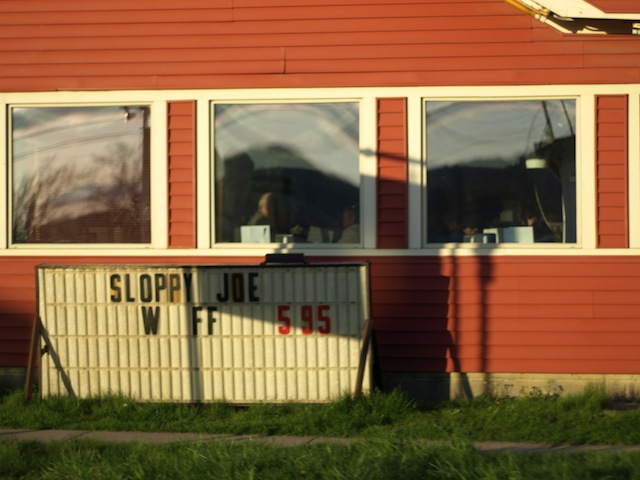The image captures the side of a red-paneled building, likely a restaurant, accented with white trim. The building has three large, square windows that allow glimpses into the interior where patrons are seated in booths. The windows are heavily reflective, showing trees, power lines, and other buildings, with notable glare from the sky. In the middle window, a person working at a laptop is visible, while the other windows show faint interior details and reflections. Below the windows on the left side, a white marquee-style sign with replaceable black letters and red numbers reads: "Sloppy Joe, W, FF, 5.95," presumably indicating a Sloppy Joe meal with fries for $5.95. The foreground is a mix of slightly overgrown grass and a gray sidewalk that stretches horizontally across the lower edge of the photograph.